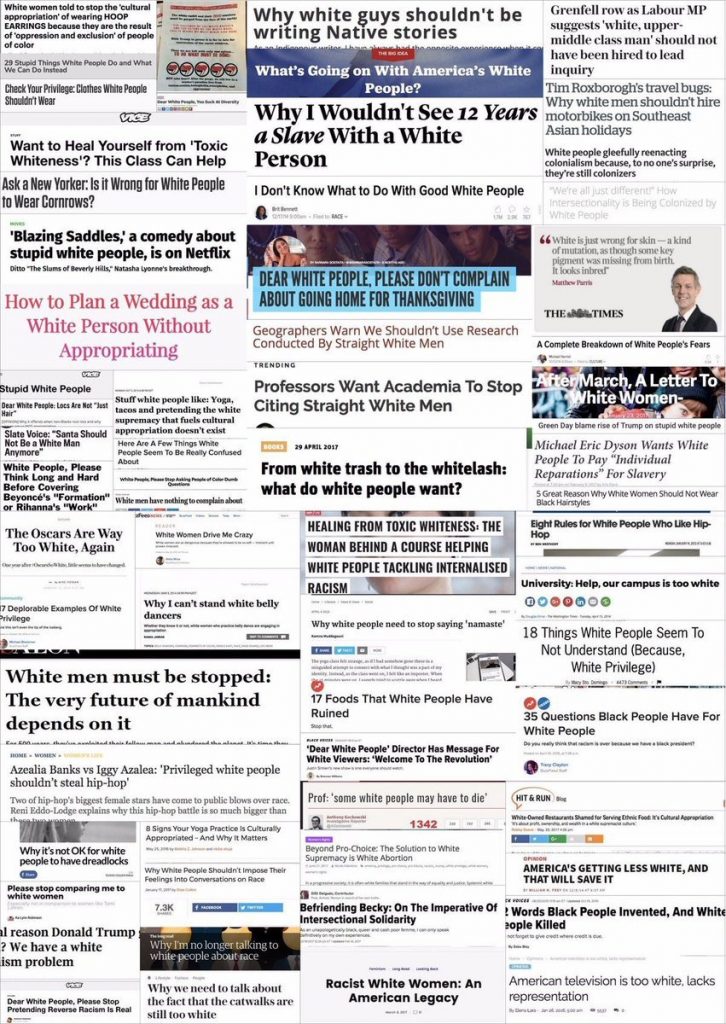This image appears to be a collage of over 30 headlines from various websites, all addressing topics related to white people. Among the headlines, you can find provocative statements and questions such as "I don't know what to do with good white people," "Why I wouldn't see 12 Years a Slave with a white person," "Want to heal yourself from toxic whiteness? This class can help," and "As a New Yorker, is it wrong for white people to wear cornrows?" 

One headline advertises the availability of the film "Blazing Saddles, a comedy about stupid white people," on Netflix, while another offers guidance on "How to plan a wedding as a white person without appropriating." Scattered among the text are images of individuals accompanied by their quotes, and in the top left corner, there appears to be a book. Above one section of these headlines is a caption: "Dear White People, please don't complain about going home for Thanksgiving."

Other notable headlines include "17 Foods that White People Have Ruined" and "Professor: Some White People May Have to Die." The visual is a striking compilation of articles and opinions, each engaging with themes of race, identity, and cultural criticism, specifically focusing on the behaviors and perceptions associated with white people.